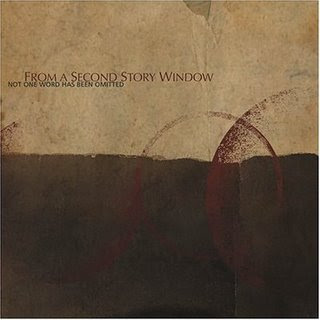This is the album cover for "Not One Word Has Been Omitted" by the band From a Second Story Window. The design is minimalist yet visually appealing. The upper portion of the cover features a light tan color that resembles the texture of aged paper. This section gradually transitions into a silhouette-like depiction of a hillside. Below this, the color shifts to a darker brown, creating a distinct two-tone effect. Scattered across the middle-right are a few red circular spots, adding a striking contrast against the more subdued background tones. The band’s name, From a Second Story Window, is printed in bold red lettering on the top-left side of the cover. Directly beneath it, the album title "Not One Word Has Been Omitted" is presented in gray lettering. Overall, the cover evokes a sense of rustic simplicity and subtle elegance.